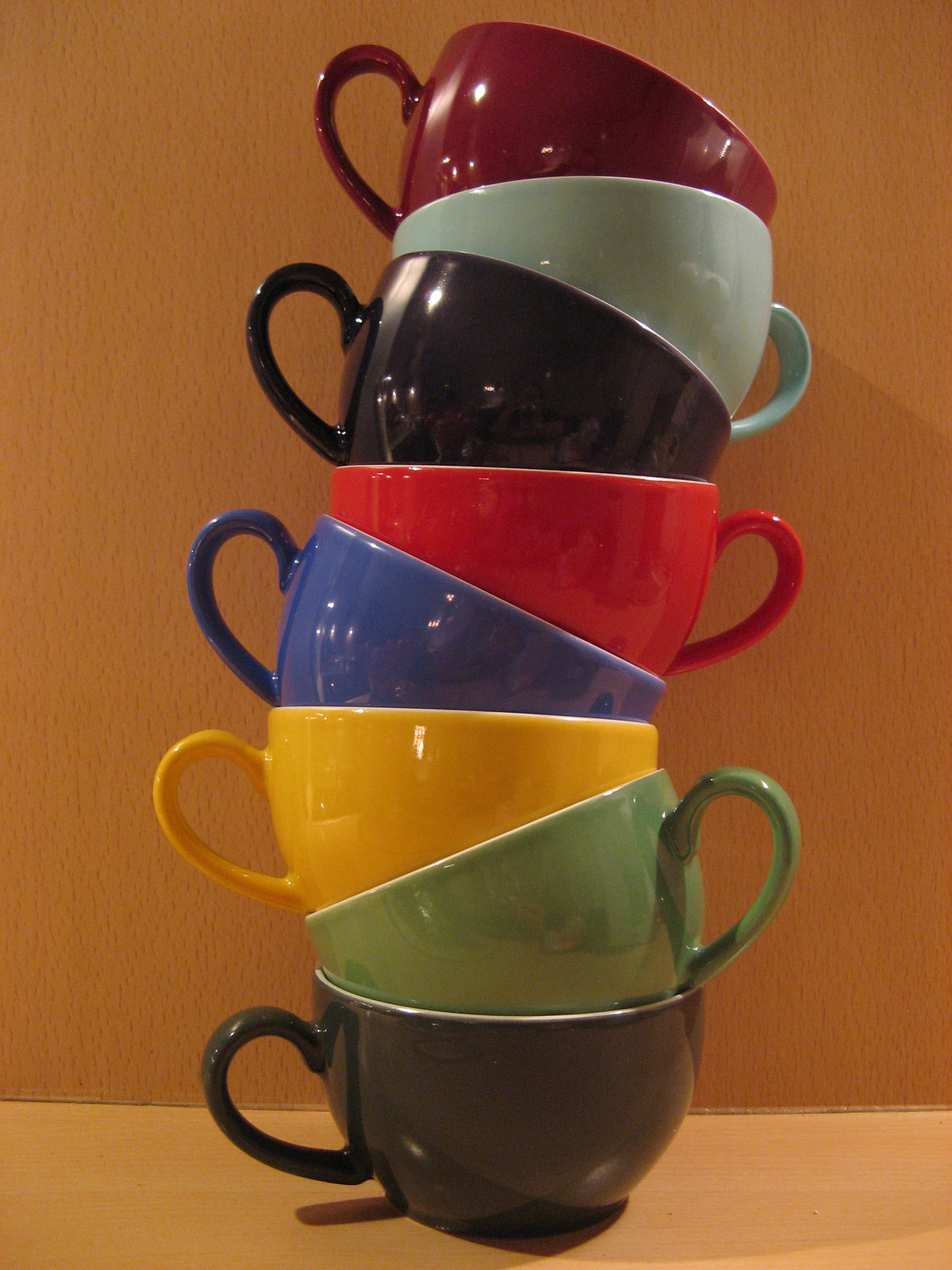The image depicts a meticulously stacked tower of round-bottomed coffee cups on a brownish-beige table with a matching background. The arrangement begins with a black-gray cup at the bottom, followed by a sequence of colors: green, sunshine yellow, dark navy blue, lipstick red, solid night black, porcelain white, and culminating with deep burgundy red at the top. The cups are systematically balanced with their handles alternating from right to left, creating a zigzag pattern that enhances the structural stability of the tall stack. Each cup reflects the ambient room light faintly, revealing some indistinct shapes like clothes on the floor, adding a subtle liveliness to the otherwise minimalist scene.